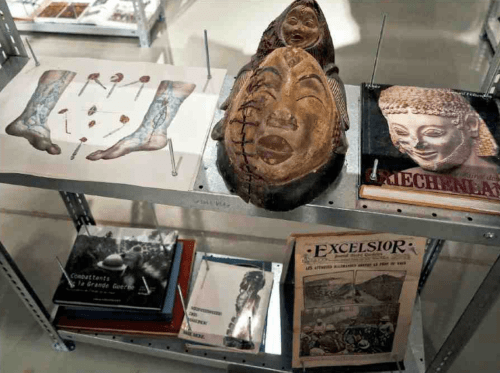This image, seemingly captured within a museum or educational center, features a detailed display on a dual-level metal bookshelf set against a concrete floor bathed in either fluorescent or natural light. The top shelf prominently displays a series of detailed diagrams on white sheets showing human feet up to the knees, depicted with veins, arteries, and additional anatomical features indicated by lines and shapes. Adjacent to the diagrams, in the center, there is a large, intricately carved wooden mask evocative of Asian art, featuring a serene face with closed eyes and pursed lips. This mask also incorporates the smaller face of an infant positioned above its head, both enveloped by a carved cloak, with a notable set of stitches resembling football laces running from the eyebrow to below the chin, possibly signifying a historic repair. To the right of this mask, there is a thick hardcover book adorned with an image of a terracotta or marble statue and indistinguishable writing at the bottom, hinting at ancient artifacts. 

On the bottom shelf, a neat arrangement of books is observed. To the left, a stack of volumes with varied colored covers – red, blue, and black-and-white – lies horizontally, topped with the image of a possibly World War I scene featuring soldiers in a trench. In the middle, more paperback books are positioned, while an upright, vertically standing newspaper with the title "Excelsior" in bold black text and a predominantly black-and-white photograph rests to the right. The photograph, despite its somewhat obscured details due to lighting glare, suggests a historical snapshot. Additional metal shelving and vague forms like books linger indistinctly in the background, enhancing the scholarly ambiance of the scene.